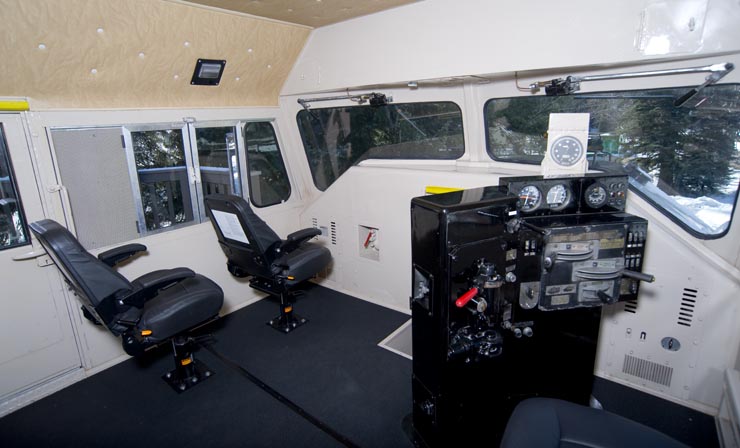This photograph captures the interior of a control room, possibly within a passenger train or a large vessel such as a boat. The front of the room features expansive windows offering a view of the outside, which appears to be high up, as evidenced by the tops of buildings seen to the right and potentially snowy trees visible in front, suggesting an elevated position, perhaps on a mountain. The room has a metallic and industrial feel with a dark floor, and the layout includes two identical black captain’s chairs bolted to the left side, one behind the other. On the right side stands a large control panel filled with horizontal metal levers, red levers, multiple gauges, and dials. These controls are essential for navigating or operating the vehicle. A small sign with the number "two" is situated atop the console. The reflections seen in the front windows hint at a nighttime setting, casting the inner part of the cabin back upon itself.